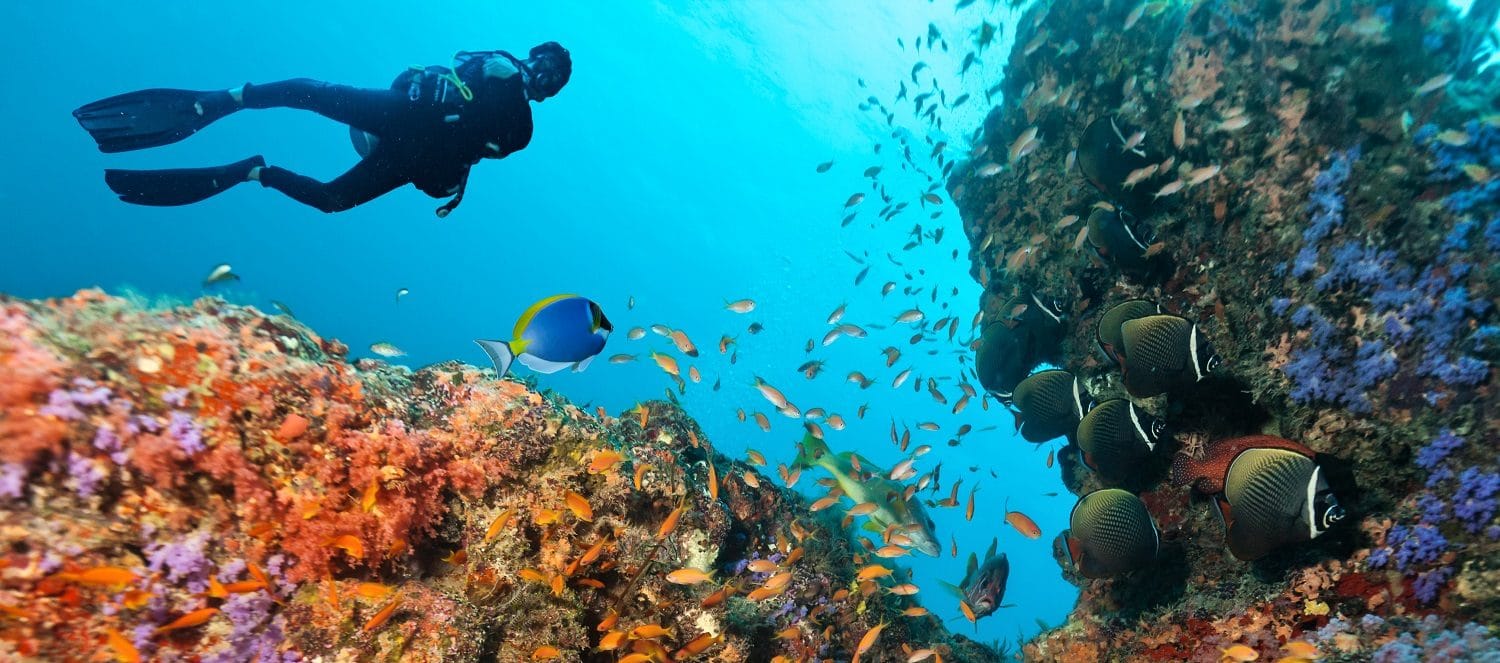This vibrant underwater photograph captures a stunning marine scene. The focal point is a scuba diver in the top-left corner, clad in a black diving suit, flippers, and face mask, with an oxygen tank strapped to their back. They are suspended in the crystal-clear, turquoise water, looking down toward the viewer with their legs extended behind them.

The bottom left corner of the image transitions to the center right, showcasing a rich tapestry of coral reefs in various shades of red, orange, purple, and blue, interspersed with rock formations. Among the reefs on the right side, flat black fish dart in and out of view, contrasting with the blue-bodied fish trimmed in yellow on the left. At the center, a plethora of tiny, minnow-like fish of different sizes cluster together, glittering in the sunlight. 

A long fish with green accents glides through the water, while another fish swims directly toward the viewer. The rest of the fish in the scene present either their sides or backs. The entire composition is a kaleidoscope of vibrant marine life against the backdrop of a thriving coral reef, illuminated by the clarity of the azure ocean water.